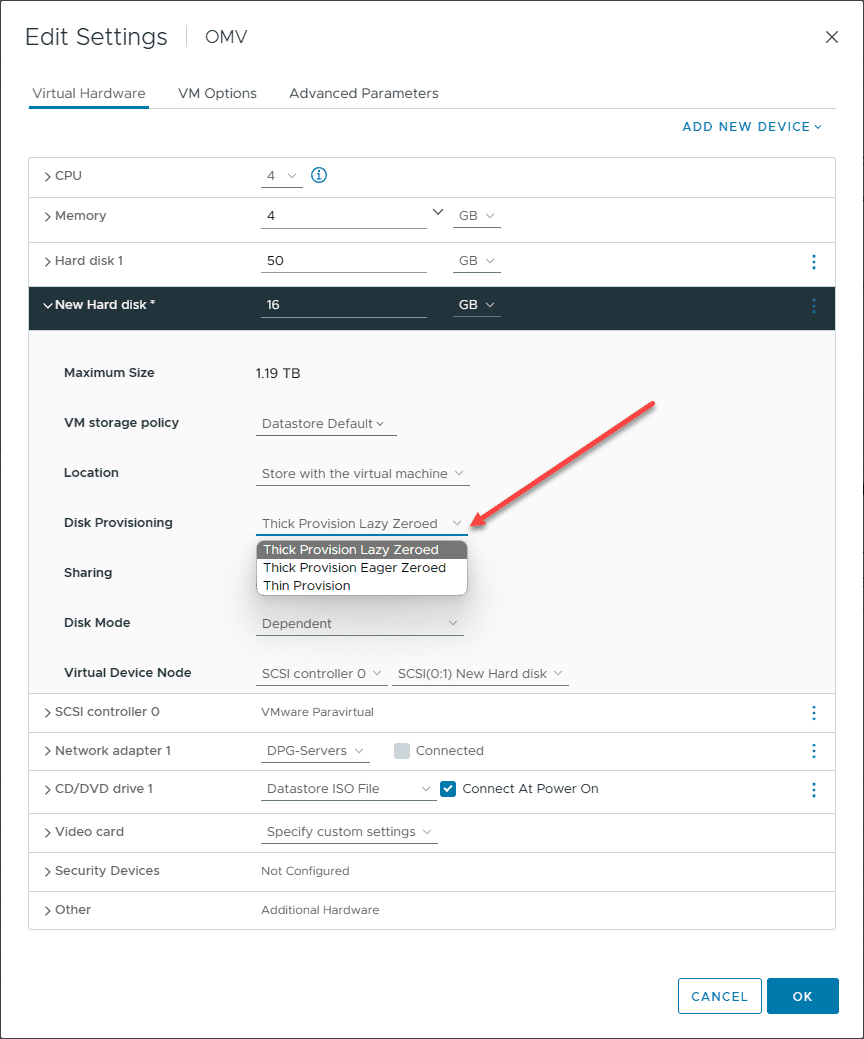Screenshot of Application Settings:  

In this detailed screenshot of an application's settings interface, the title "Edit Settings" is prominently displayed in the top left corner. A bar labeled "OMV" lies beneath it, while an X button for closing the window is situated in the top right corner. The interface is divided into three tabs: "Virtual Hardware" (currently selected, indicated by a blue underline), "VM Options," and "Advanced Parameters." 

Below the tabs on the right side, there's blue text labeled "Add New Device" with a dropdown arrow beside it. This area categorizes various settings: 

- **CPU:** Set to four.  
- **Memory:** Set to four gigabytes.  
- **Hard Disk 1:** Configured to 50 gigabytes.  

The current selection is focused on a navy-boxed option related to a new hard disk set at 16 gigabytes. 

Additional information is displayed regarding:
- Maximum Size
- VM Storage Policy
- Location
- Disk Provisioning
- Sharing
- Disk Mode
- Virtual Device Node

An arrow highlights the expanded dropdown menu for Disk Provisioning, showing the selected option "Thick Provision, Lazy Zeroed" in a gray box. Other available options include "Thick Provision, Eager Zeroed" and "Thin Provision."

Further configuration categories are listed below:
- **SCSI Controller 0:** Set to VMware ParaVirtual.
- **Network Adapter 1:** Set to DPG servers, with the adjacent "Connected" checkbox unchecked.
- **CD/DVD Drive 1:** Set to Data ISO File, with the checkbox checked to enable "Connect at Power On."
- **Video Card**
- **Security Devices**
- **Other**

In the bottom right corner of the interface, there are two buttons: a white button with blue text labeled "Cancel" and a larger blue button labeled "OK."